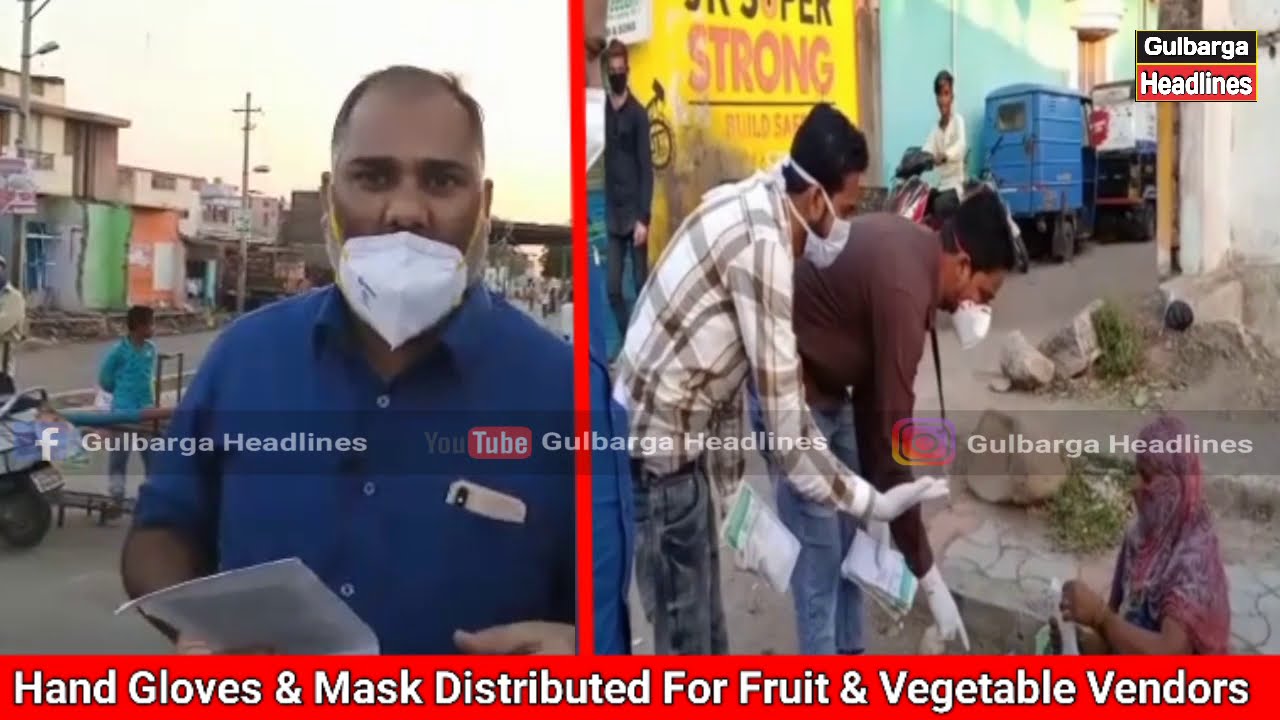This still image from a newscast is divided into two side-by-side pictures, each illustrating a scene on a street in a developing country. On the left side, a man with brown skin, dressed in a blue shirt and wearing a white COVID-19 face mask, stands facing the camera, holding a paper in his hands. The background reveals an urban setting with roads, vehicles, and houses, exhibiting a somewhat dilapidated appearance. On the right side, an elderly woman with a headscarf is seated on the ground, while two men, also wearing COVID-19 face masks and gloves, stand bending over her as if offering assistance, possibly giving her instructions or distributing items. The background here also shows vehicles, people, and older buildings. In the top right corner of the image is the logo "Gulbarga Headlines." A red strip runs along the bottom with the text "hand gloves and masks distributed for fruit and vegetable vendors." A transparent strip watermark across the middle of the image features the "Gulbarga Headlines" logo accompanied by Facebook, YouTube, and Instagram icons.